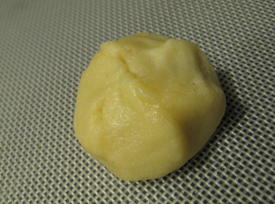In the small, rectangular image, there is a close-up photograph of a yellowy cream-colored ball of dough, most likely cookie dough, resting on a surface that resembles a wire crisscrossing pattern. The background is black and white, appearing like a screened or metallic pan. The dough has a smooth but worked texture, with visible hand markings and indentations, indicating it has been rolled and shaped by hand. The dough ball is roughly formed, not perfectly round, with a noticeable split at the top where it appears folded together. There is a shadow cast to the right of the dough ball, suggesting the light source is from the left.